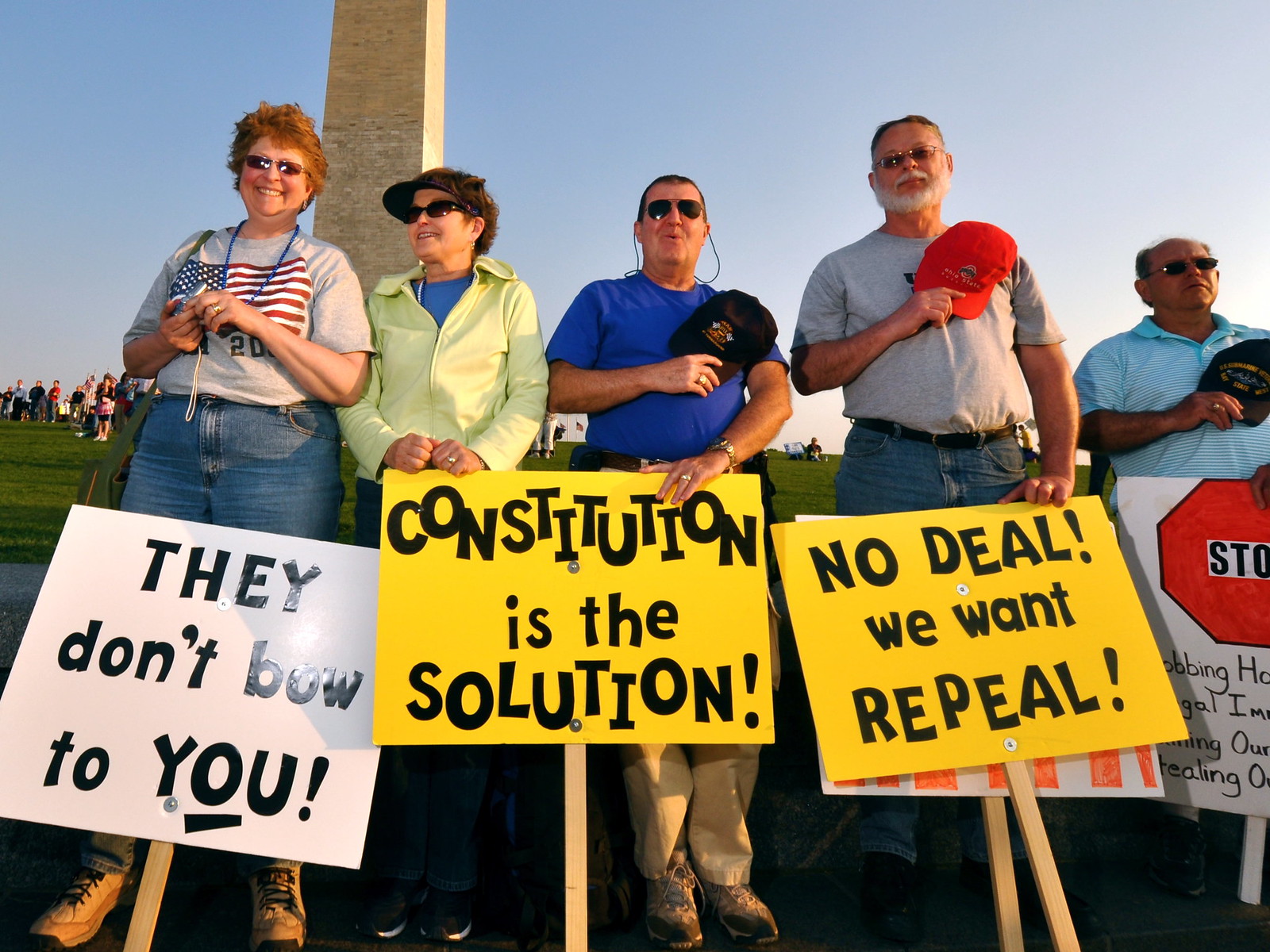This color landscape photograph captures a group of five elderly individuals posing in front of the Washington Monument, possibly during a protest. The group stands side by side, with three men on the right and two women on the left. All five individuals are dressed in casual clothing and wear sunglasses. Notably, the three men are holding their ball caps over their hearts in a gesture akin to a salute, while the women look directly toward the viewer with smiles. Each person holds a sign: the woman on the far left holds a white sign reading "They Don't Bow to You" in black lettering; the individuals in the center display a yellow sign with the message "Constitution is the Solution!" in black letters; the man on the right holds a yellow sign that reads, "No Deal! We Want Repeal!" in black letters. Behind them, more people and the towering Washington Monument are visible, under a blue sky hinting at late evening, as suggested by the long shadows cast to the left. The scene encapsulates a moment of peaceful protest and patriotic expression.